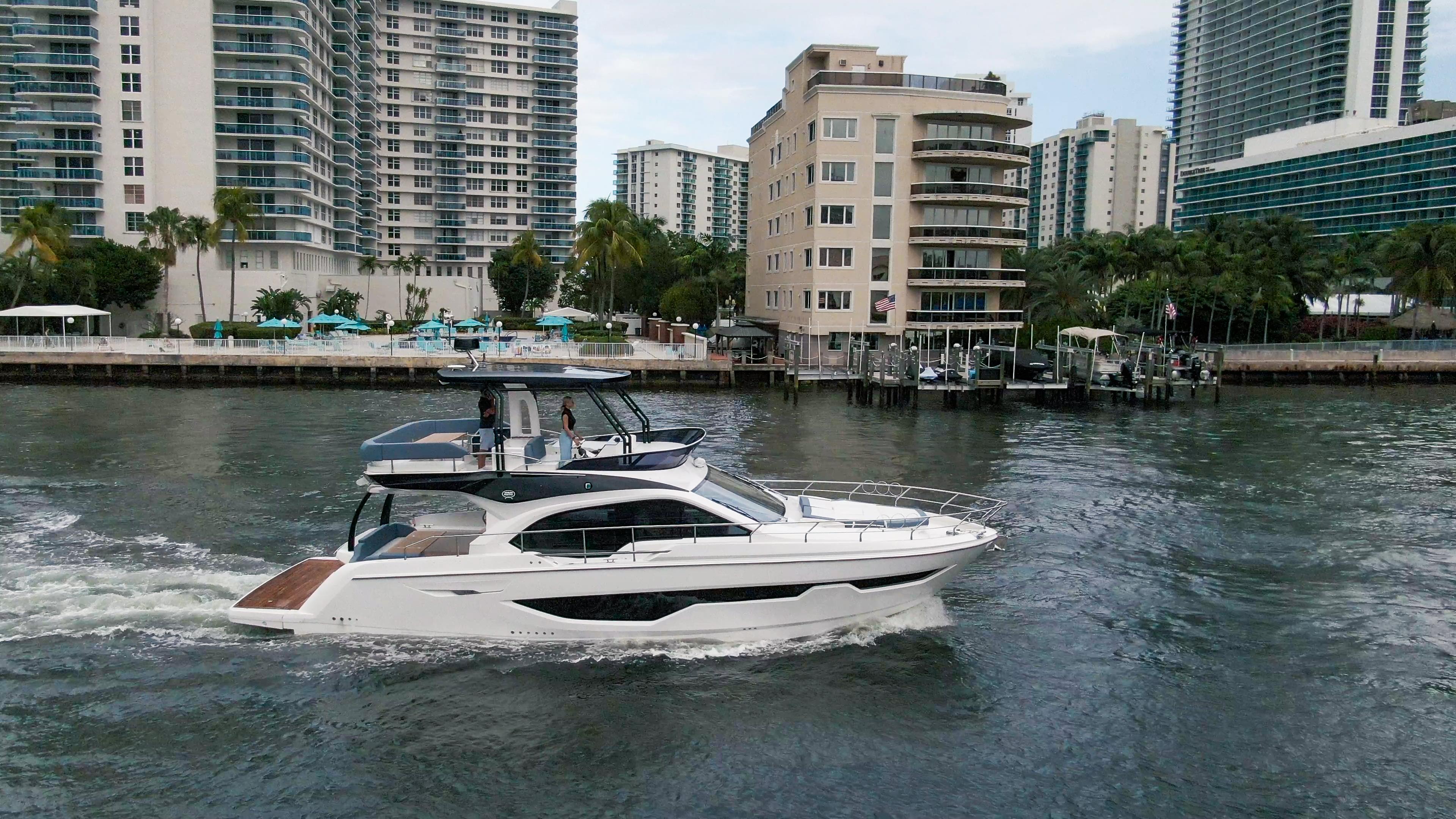This image captures an outdoor scene in a harbor under a blue sky dotted with gray clouds. A white motorboat, possibly a small yacht, is prominently featured as it moves from left to right across dark gray waters, leaving a churning, greenish-white wake behind it. The boat has a bottom cabin area with tinted black windshields and a central section topped by a piloting area. A woman of Caucasian descent, dressed in a black shirt and blue pants, stands confidently at the steering wheel on top of the cabin. Behind her, a man in blue shorts and a black shirt is visible. The boat also features a small swimming platform at the back.

The background reveals a bustling harbor scene with several other boats docked along a boardwalk. Dominating the skyline are multi-story buildings with balconies, potentially apartments or condominiums. To the left, a towering structure rises about 20 stories high, accompanied by a shorter, five-story brown building adorned with an American flag. A gray building is situated in the top right-hand corner of the image. The dock area is lively, featuring outdoor umbrellas, tables, and chairs, and dotted with a few palm trees, further enhancing the resort-like atmosphere of the scene.